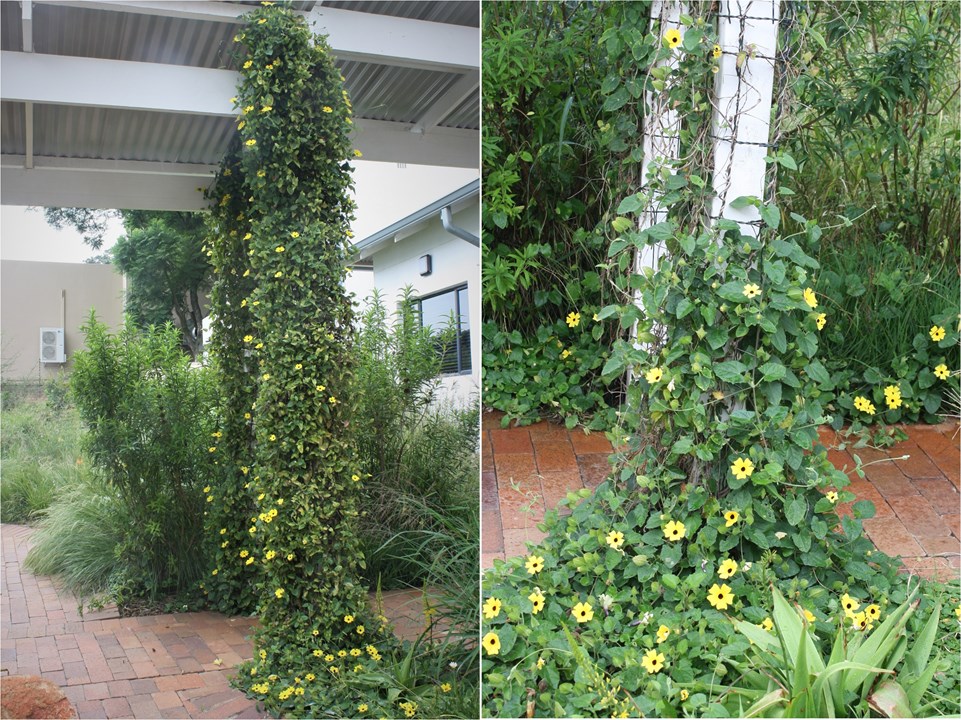The image is a collage featuring two outdoor photos of the same setting. The left photo shows an archway adorned with green plants and vibrant yellow flowers, situated under a metal ceiling akin to a roofed deck. The archway stands on a red brick pathway with a white, one-story house in the background to the right, featuring a gutter pipe. A brown building with what appears to be a heating unit is partially visible in the distant background.

In the right photo, the focus is on a lush cluster of yellow flowers and green plants, climbing up the lower portion of the same archway from the previous image. The upper part of the arch is less covered. The scene also features additional yellow flowers to the right, green bushes in the backdrop, and the red brick pathway seen in the left photo. Both images are text-free and showcase a slightly overgrown yet charmingly natural garden area.